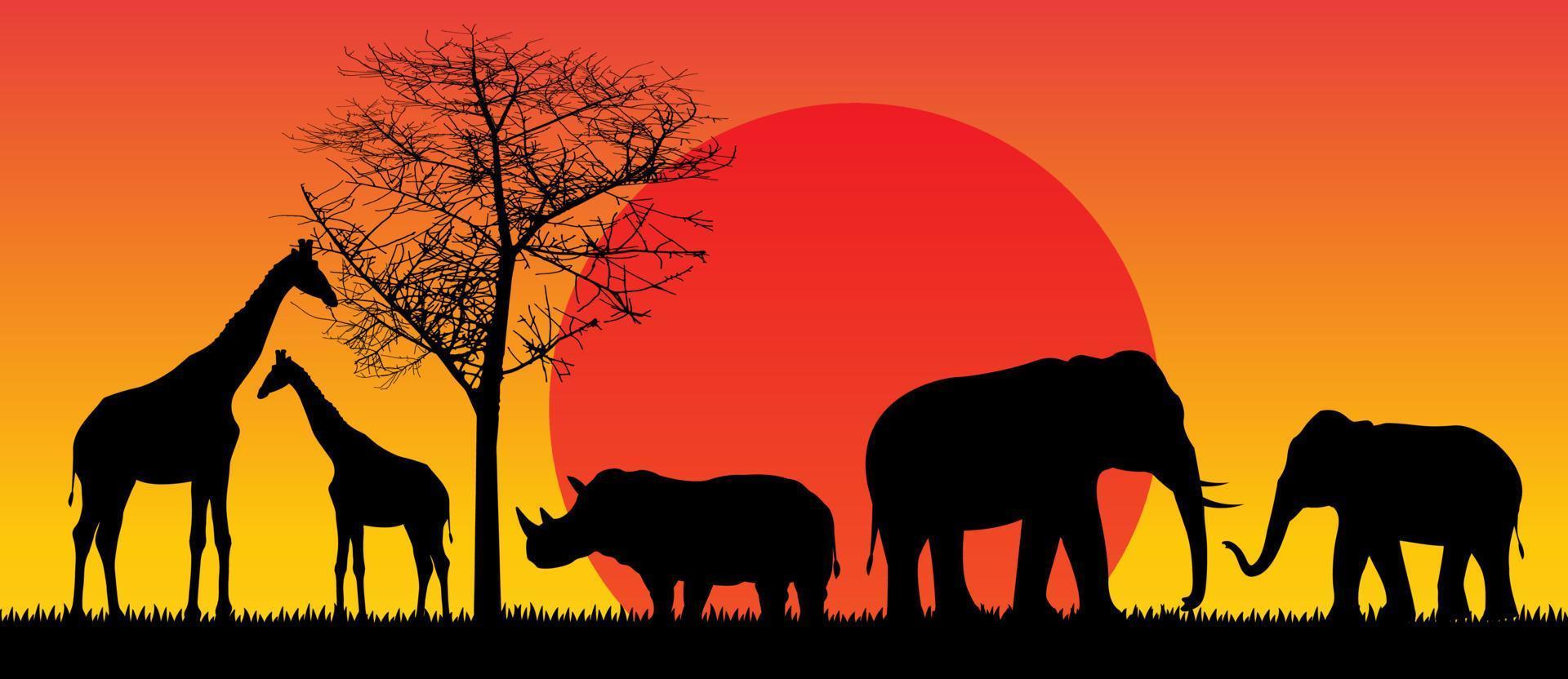The image showcases a vibrant sunset scene with an orange and yellow gradient sky, and a large red sun positioned in the middle. The scene is set against a silhouette of African wildlife, all depicted in black against the bright background. Dominating the left side of the image is a tall, leafless tree reaching to the height of the picture. Standing in front of the tree are two giraffes—one tall and another shorter—facing each other. To the right of the tree is a rhino, also in silhouette, facing towards the giraffes. On the extreme right side of the image, there are two elephants: a larger elephant with tusks, and a smaller, tuskless (or minimally tusked) baby elephant. Both elephants are positioned to face each other. The ground and grass are indicated with a black outline beneath the animals, continuing the silhouette theme. The detailed contrasts and arrangement of the animals against the fiery backdrop capture the essence of an African sunset, bathed in warm orange and yellow hues.